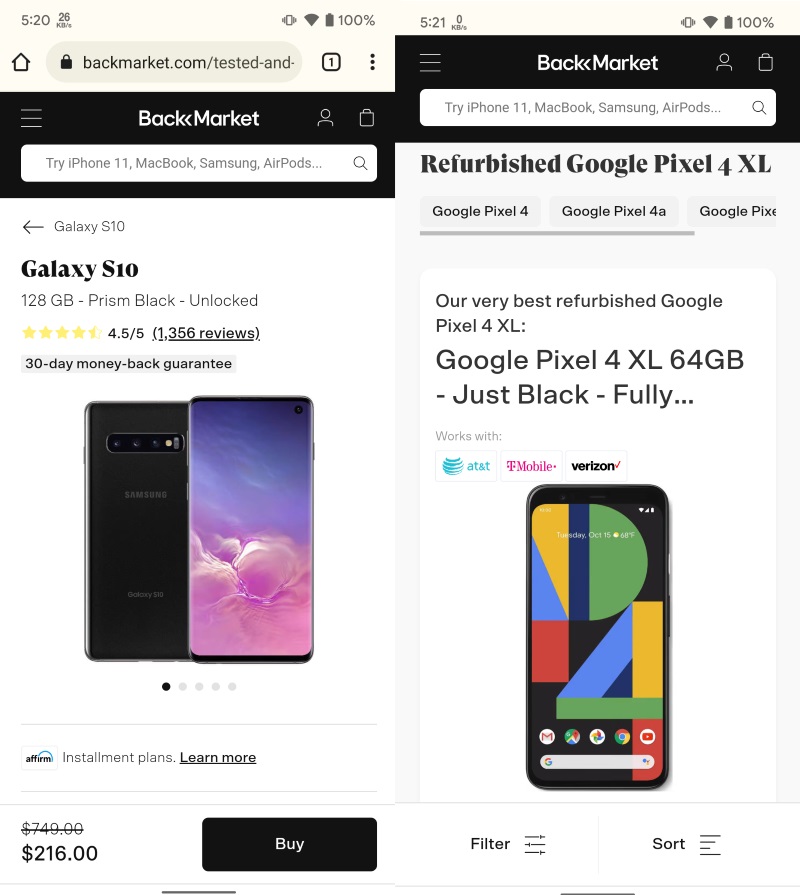In the pair of screenshots from the website Backmarket.com, an individual is searching for a new cell device. The search bar at the top indicates the query, leading to two specific listings.

On the left side:
- The listing features a Samsung Galaxy.
- It is a refurbished device with a storage capacity of 128GB, in prism black color, and unlocked.
- Reviews are available for further reading.
- The device is priced at $216, with Affirm offered as an installment payment option.
- The "Buy" button is prominently highlighted in black.

On the right side:
- The listing shows a refurbished Google Pixel 4XL.
- It offers a storage capacity of 64GB and is labeled as "very best refurbished."
- The listing includes a picture of the phone displaying a Google screen with the model abbreviation "P4."
- At the bottom, there is a filter and sort menu, allowing users to refine their search further.

Overall, the screenshots collectively display the different options available for refurbished phones, highlighting key details such as price, conditions, and purchase options.